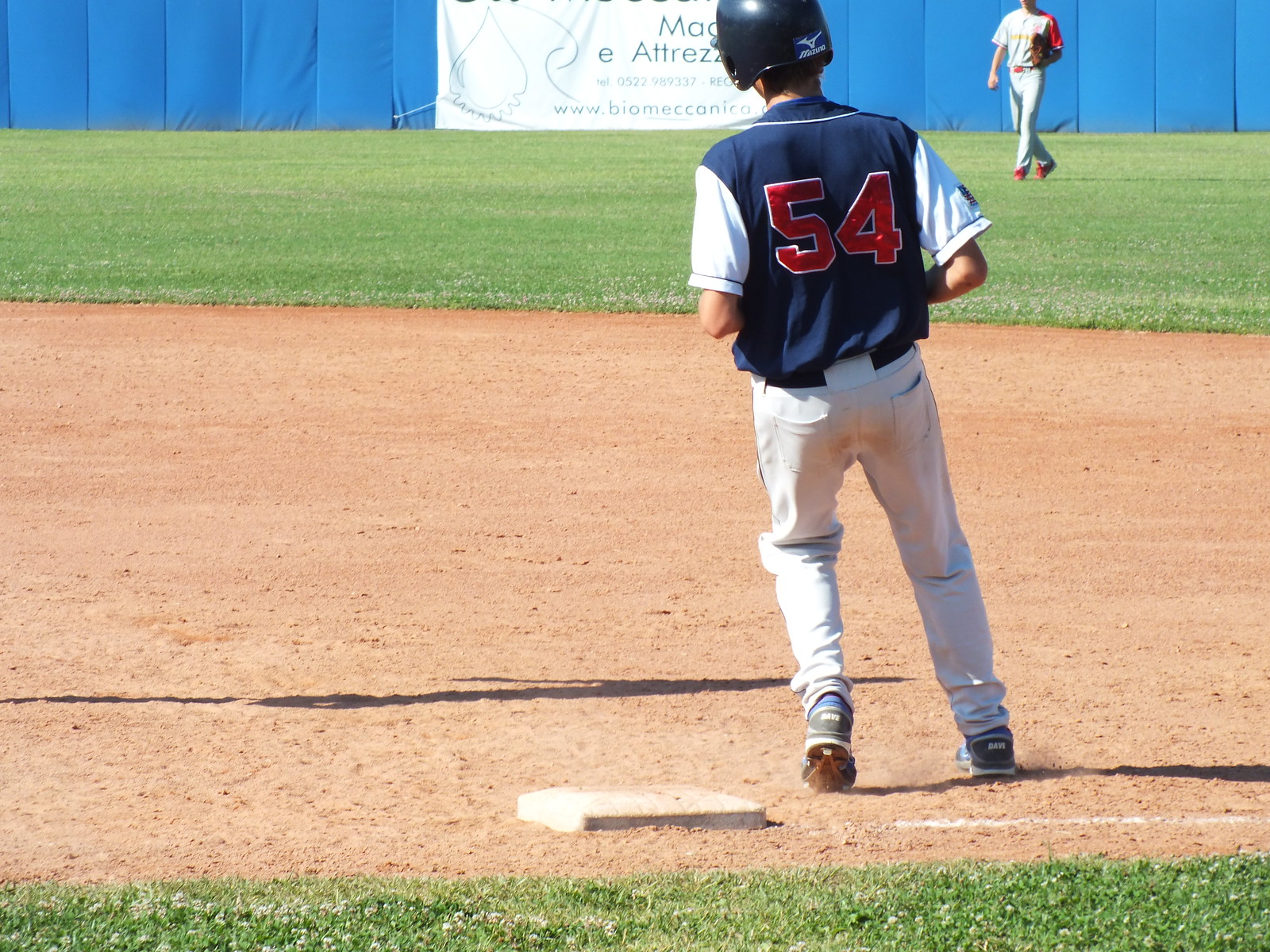This image captures a dynamic moment in a baseball game, with the main focus on a player who appears to be assessing his next move. The player, standing on a dirt infield with meticulously maintained green grass around him, is clad in a blue jersey with white sleeves and the number 54 in red on his back. He wears long white baseball pants, cleats, and a dark helmet, and appears to be looking toward another player in the outfield. The outfield player, partially obscured and donning a gray uniform, is positioned near a blue fence adorned with a white advertisement sign. The field is neatly divided with green grassy areas and a light tan infield, showcasing a well-maintained sports venue. The scene suggests a pause in the action, perhaps after an overrun base, with the focal player standing beside a white base in the lower center of the image.